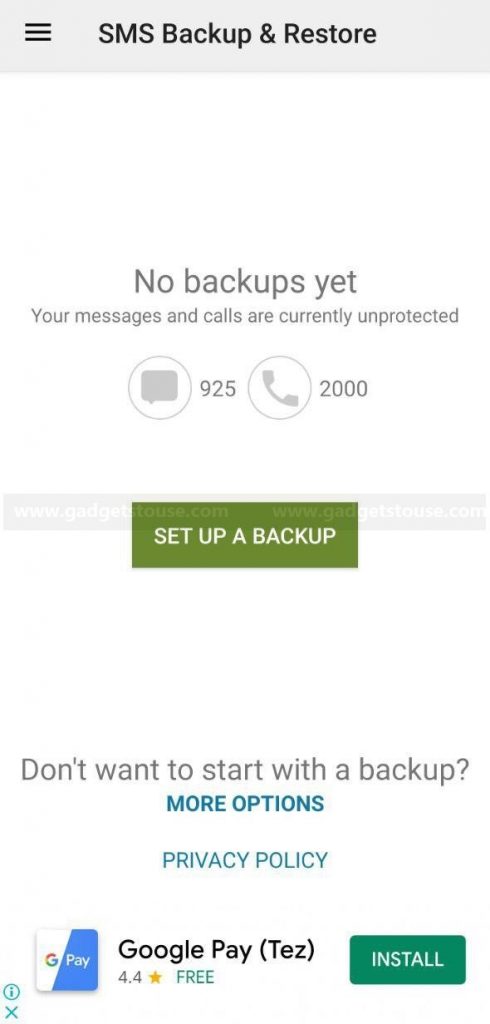Screenshot Description: 

The screenshot captures a mobile phone interface, predominantly featuring a clean white background. At the top, a light gray bar spans horizontally across the screen, approximately one inch in height. Situated in the top-left corner within this gray bar are three horizontal black lines, each around half an inch long, stacked one above the other.

Centered below the gray bar in large, bold, black capital letters are the words "SMS BACKUP & RESTORE." Beneath this, there is a gap of about two inches, followed by the text "No backups yet" in a faded black font. Directly under this, in smaller lettering, it states, "Your messages and calls are currently unprotected."

Further down, the interface features two white circles, each with a gray border. The first circle contains a gray speech bubble icon, accompanied by the number "925" to its right. The second circle to the right of the first displays a gray phone icon, with the number "2000" beside it.

Below these icons is a prominent green pop-up tab with white text that reads "Set a backup." Beneath this, in black text, it asks, "Don't want to start with a backup?" 

Following this question, in teal green all-capitalized bold letters, it reads "MORE OPTIONS." Below this in regular teal lettering is "Privacy Policy," also capitalized.

In the bottom-left corner of the screenshot, there is a small blue "X" icon. Above this, there's a circular icon with a blue border containing a small letter "i." 

Adjacent to these elements, on the right side, appears a square divided into two halves: the left half is white with the classic Google "G," and the right half is blue with the word "Pay" in white. To the right of this square, in small black text, are the words "Google Play (Tez)" followed by a rating of "4.4 stars" in black text. Below this, in all-capitalized green letters, it says "FREE."

Finally, in the bottom right corner, there is a green or teal green tab with white text that reads "INSTALL."